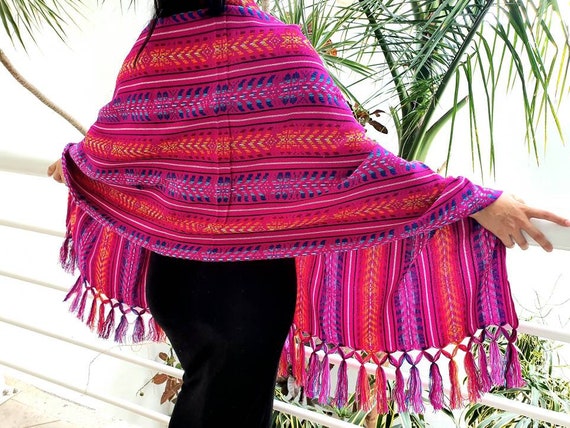In this outdoor photographic image, a woman with long black hair is positioned with her back to the camera, standing at a white railing, her hands lightly gripping it. Dressed in a long black dress that reaches down to her knees, she is enveloped in a wide, multicolored scarf that drapes down to her waist. The scarf boasts a palette dominated by purples, reds, oranges, and a touch of pink, arranged in seven or eight chevron-style bands. The scarf’s bottom edge is adorned with fringes in matching colors. Although her face is not visible, her pale arms and the tops of her legs are. Set against a backdrop of a palm tree and a bright sky, the woman's stillness and the vivid colors of her scarf make for a striking contrast, suggesting a moment of quiet contemplation in a sunlit, plant-filled environment.